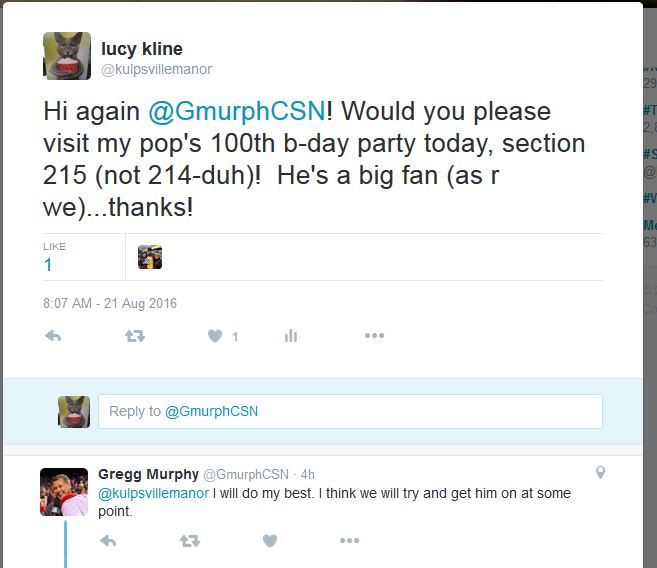This image is a detailed color screenshot of a social media post from the old Twitter interface, dated August 21st, 2016, at 8:07am. The post is by Lucy Klein, whose handle is @KULPSVILLEMANOR, and it features a color icon of a cat holding a red object. The message reads: "Hi again @GmurphCSN. Would you please visit my pop's 100th birthday party today? Section 215. Not 214, duh. He's a big fan, as are we. Thanks." The post received one like and displays the tag information and username beside the cat icon. Below the original post, there is a reply by Greg Murphy, whose handle is @GmurphCSN, accompanied by a photo of a smiling man in a crowd. His response reads: "I will do my best. I think we will try and get him on at some point." The screenshot is in a square format and showcases the typical social media conversation style with icons, reply bars, and comments.